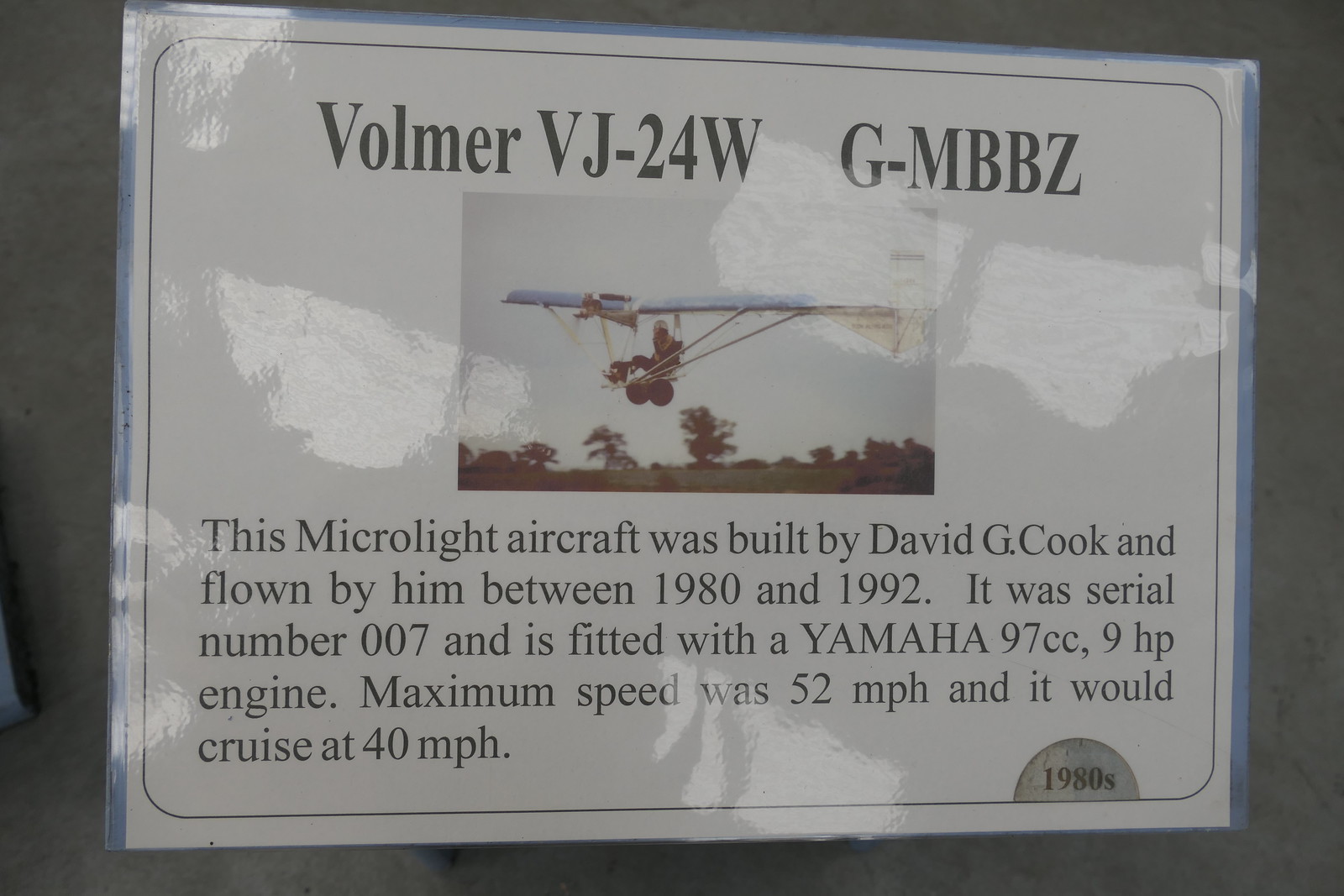This detailed photograph showcases a laminated sign on white paper featuring a historical microlight aircraft. The sign, bordered by a black rounded edge frame, includes a color photograph of the Vollmer VJ-24W aircraft, registration G-MBBZ. The image depicts an individual wearing a helmet seated in the aircraft, which has wings above, wheels beneath, and offers a clear view of the ground, sky, and a few trees in the background. Above the photograph, the text reads "Vollmer VJ-24W GM BBZ." Below the image, a descriptive passage states: "This microlight aircraft was built by David G. Cook and flown by him between 1980 and 1992. It was serial number 007 and is fitted with a Yamaha 97cc 9 horsepower engine. Maximum speed was 52 miles per hour and it would cruise at 40 miles per hour." In the bottom right corner of the sign, the text "1980s" is inscribed within a gray semicircle, suggesting an organization by decades, possibly for display in an aviation museum.